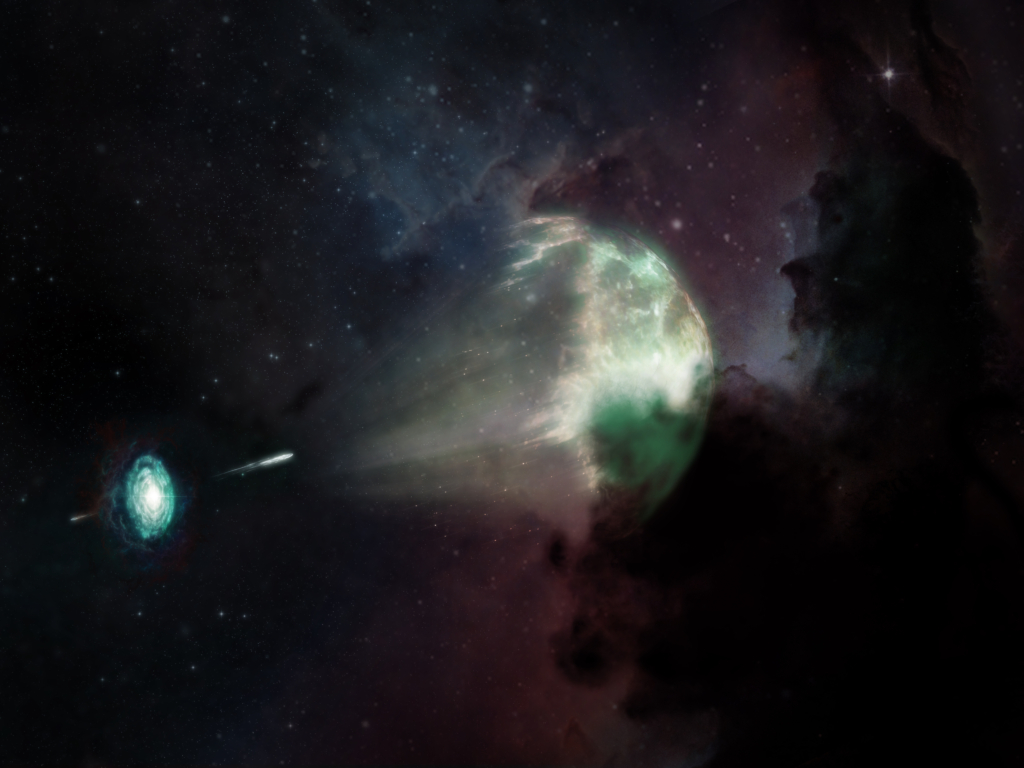This rectangular, landscape-oriented, space-themed illustration, measuring approximately six inches wide and four inches high, portrays a captivating outer space scene. Dominated by a central glowing light, the composition seems to depict a dynamic event such as space travel, a comet, or perhaps an encounter with a UFO.

In the foreground at the lower left corner, a small satellite or circular object, colored aqua blue or green, appears to be launching a missile-shaped projectile or emitting a bright, thin, diagonal trail of light. This trail crosses over the scene, leading towards the center-right area of the image where it intersects with the central glowing light source.

The central light source is depicted as a bright, oblong circle with a blue ring encasing a radiant white core, framed by black and dark green clouds. This light creates an intense visual contrast, casting rays that illuminate the surrounding galactic formations and constellations.

In the background, the illustration showcases the iconic M42 nebula from the constellation Orion, depicted with vibrant hues; to the right are striking pink clouds and to the left, transitioning from black to blue, are grayish-blue gaseous formations. There are also notable black clouds with a red tinge in the background on the right-hand side. The entire scene is set against the backdrop of a star-studded, black cosmos, with a transparent shadowy layer adding depth and intrigue to the illustration.

It's a detailed and vivid space art piece that vividly captures the suspense and beauty of an interstellar event.